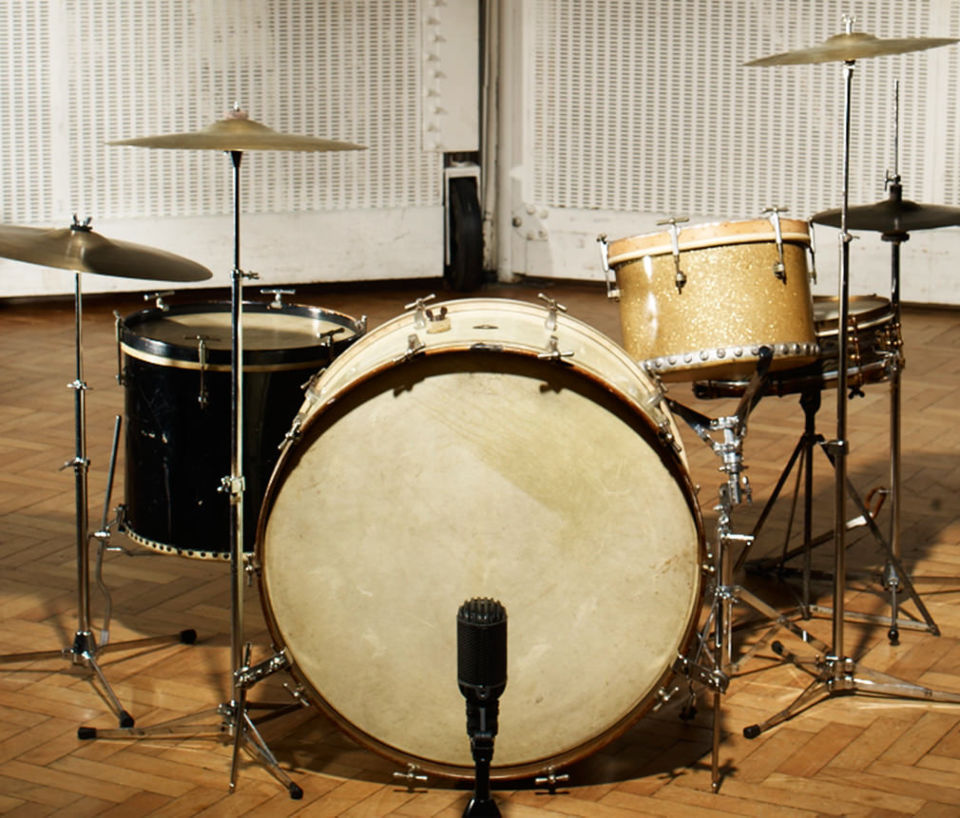This image showcases a drum set situated on a light brown parquet wood floor, presented in a predominantly square but slightly horizontal photograph. Central in the frame sits an off-white or cream-colored large bass drum, flanked by a small black snare drum to its left and a smaller tilted gold-colored drum on a stand to its right. Each side of the drum set features two cymbals mounted on stands. A black microphone is positioned directly in front of the large bass drum, hinting at a setup designed for sound recording. The background comprises white elements that seem like soundproofing material, although specific details are unclear due to the image's close-up nature. There are no visible performers or textual elements in the image, emphasizing the drum set, which appears meticulously arranged and ready for use in an indoor music room. Colors across the scene include shades of brown, beige, tan, white, black, silver, and gray.